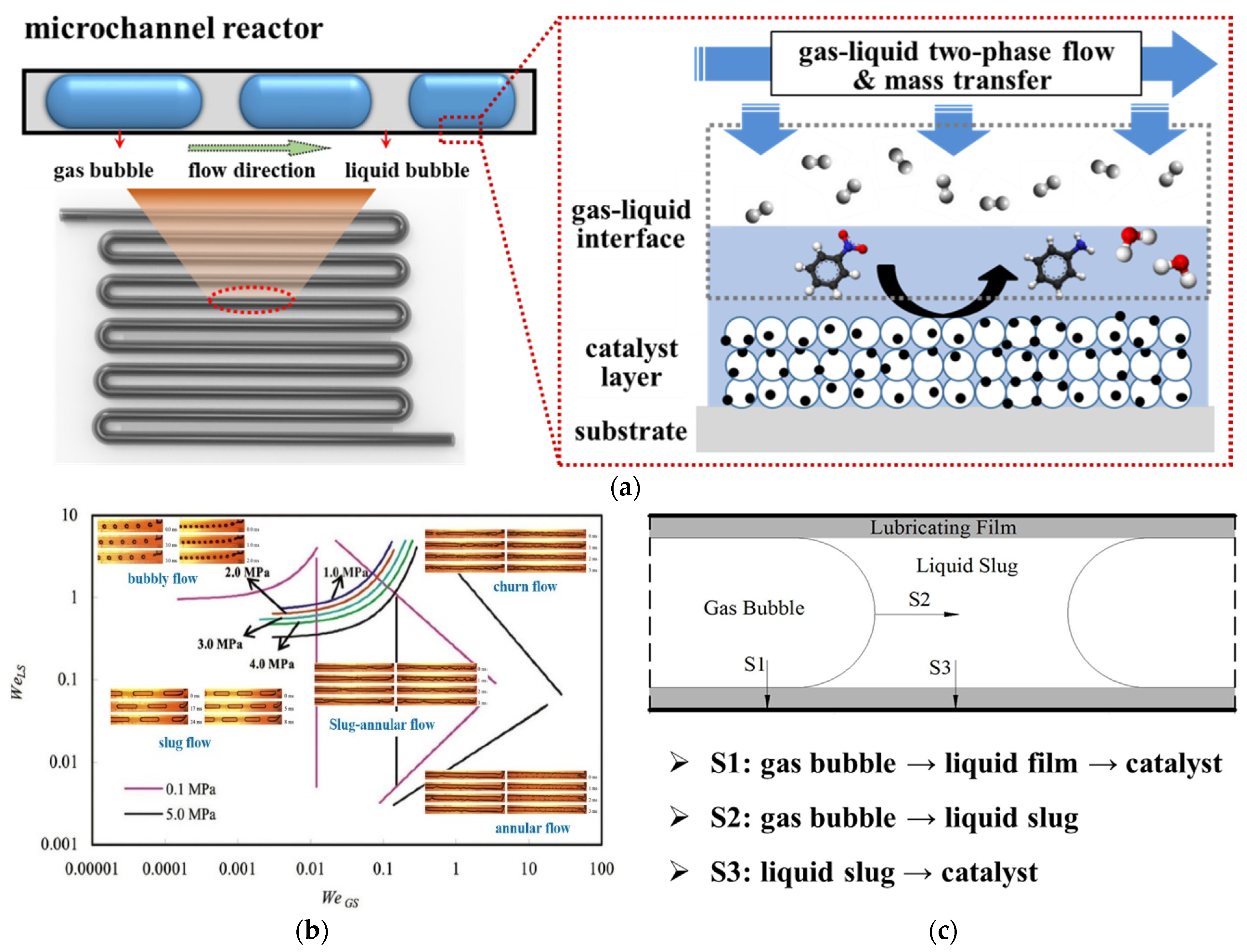The image is a detailed scientific diagram divided into four quadrants, primarily illustrating a microchannel reactor and its processes. The top left section is labeled "Microchannel Reactor" in black text and features two oblong, pill-shaped objects labeled "Gas Bubble," "Flow Direction," and "Liquid Bubble." Below these objects is a zigzagging gray piping structure spanning six levels, indicating the flow pathways. 

The top right quadrant displays a schematic titled "Gas-Liquid Two-Phase Flow and Mass Transfer," with blue arrows pointing left to right and downwards, demonstrating the directional flow. It includes annotations for "Gas-Liquid Interface," "Catalyst Layer," and "Substrate." 

In the lower left, there is a chart labeled with different flow regimes: "Bubbly Flow," "Churn Flow," "Slug Flow," "Annular Flow," and "Annular Flow" again, indicating the different phases of gas-liquid interactions. 

The lower right quadrant contains another diagram within a rectangular frame, detailing "Gas Bubble," "Liquid Slug," and "Lubricating Film," with three lines labeled "S1: Gas Bubble to Liquid Film to Catalyst," "S2: Gas Bubble to Liquid Slug," and "S3: Liquid Slug to Catalyst," highlighting the various stages of interaction and film behavior. The layout is horizontally oriented, showcasing a cohesive flow from one segment to another, effectively modeling the transformation of gas to liquid within the reactor.